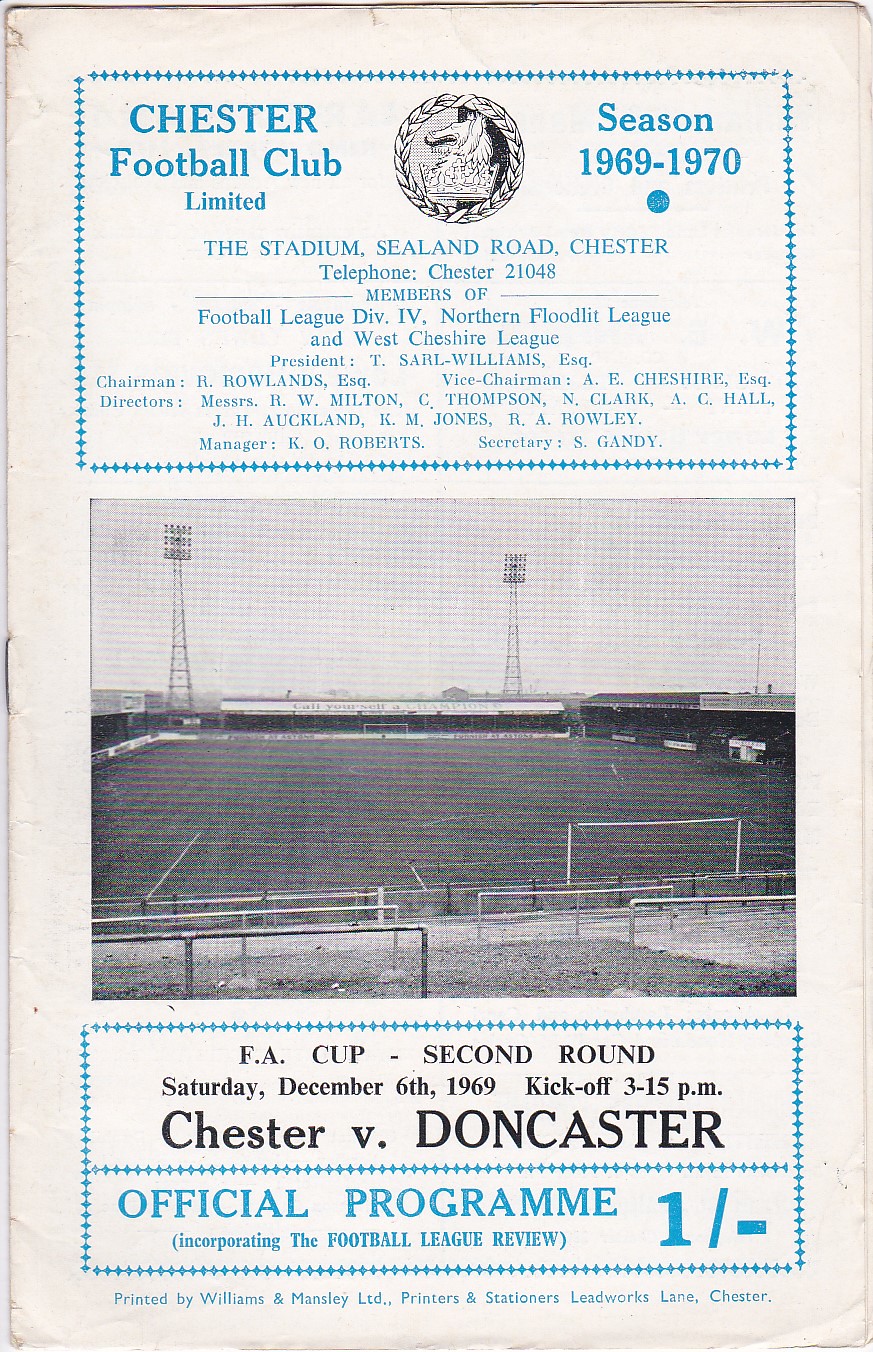This image is an aged off-white newspaper advertisement or official program for Chester Football Club, dating from the 1969-1970 season. At the top center, a black square features the heading "Chester Football Field." To the right, blue text denotes the season "1969 to 1970." Below the heading, small detailed blue text provides club information, though it’s hard to read. Centrally placed is a black-and-white photograph of the football stadium, showcasing the field, large lights in the background, and goalposts with a railing in the foreground. Below the photo, another blue rectangular box contains the details of the FA Cup second-round match on Saturday, December 6th, 1969, with kickoff at 3:15 p.m., featuring the game between Chester and Doncaster. The final lines in blue text confirm this as the official program, incorporating the Football League Review.